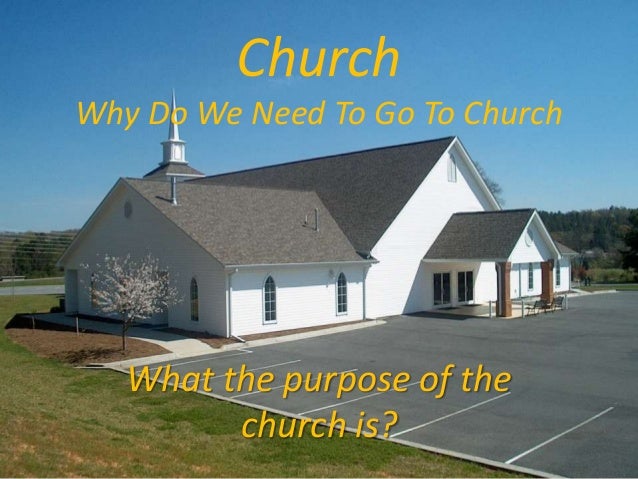This photo captures an outside view of a white church with a gray roof and a small steeple visible in the background. The church is fronted by an empty asphalt parking lot marked with white lines and features two rustic orange or brown cement brick pillars. To the left of the church, there's a grassy, hilly area that includes a tree with white leaves and flowers, as well as additional trees and shrubbery in the background. The sky is a clear blue, indicating a daytime setting. Yellow text is centered at the top of the image, reading "Church: Why do we need to go to church?" At the bottom, it continues with "What is the purpose of the church?" The photo captures the tranquil atmosphere and landscaping surrounding the church, highlighting the inviting yet contemplative setting.